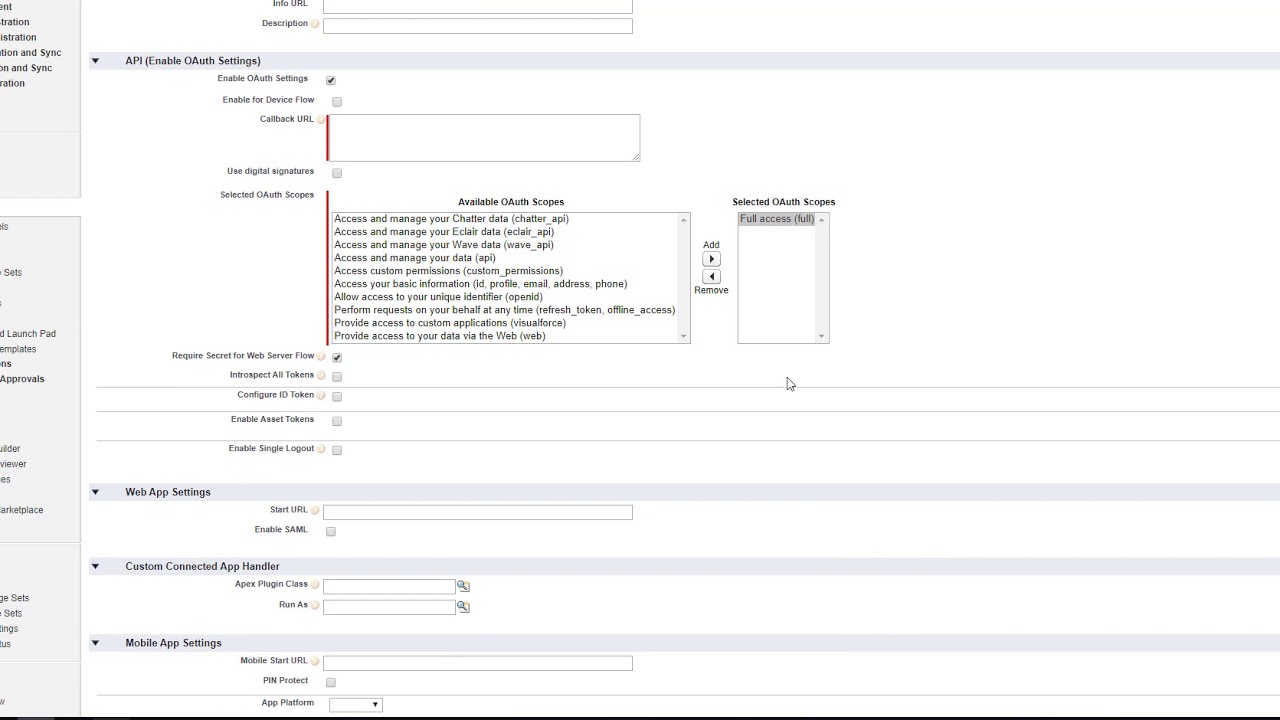This image appears to be a screenshot of a web page interface, likely part of a developer's console or a settings page for configuring application settings, with a predominantly white background and black text. 

At the top, there is an "Info URL" label accompanied by a text box where an URL can be entered, followed by a "Description" label with another text box for input. Below these, a blue line separates the segments, inside which it reads "API Enable A, A Off Settings." 

The section below this blue divider includes more configuration options represented with black text and various input boxes. Prominent labels include "Callback URL," "Use Digital Signature," and "Selected OAuth Scopes." A larger rectangular box labeled "Available OAuth Scopes" lists multiple selectable options. One of the checkboxes labeled "Require Secret for Web Server Flow" appears to be selected. 

Further down, there are labeled sections for additional configurations such as "Web App Settings" with its corresponding input box, and "Custom Connected App Handler" with multiple fillable fields.

At the bottom, a section titled "Mobile App Settings" is followed by another text input box. The left margin of the image contains a vertical strip of grey with partially visible black text, possibly indicating that part of a side menu or another segment of the page has been cut off from this screenshot.